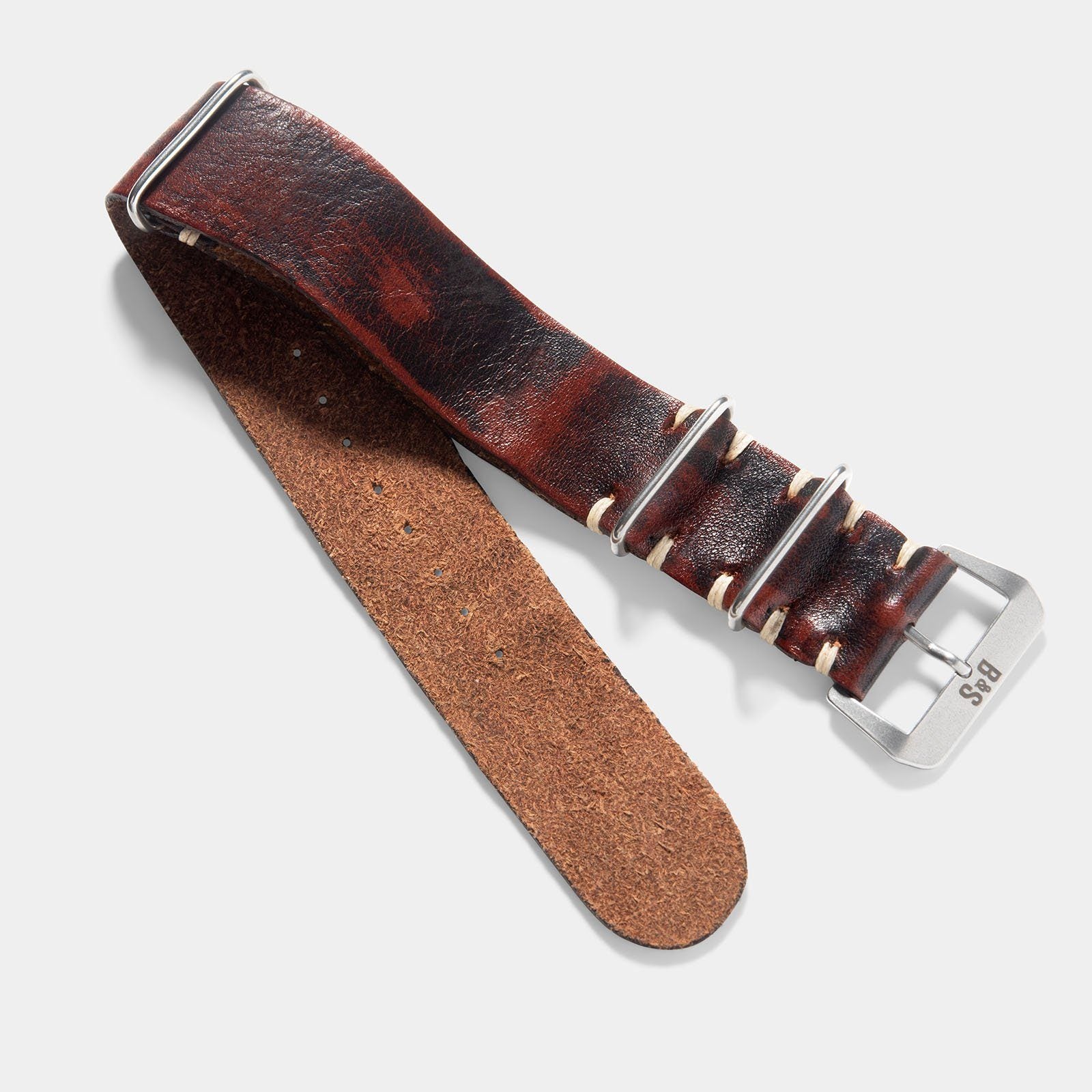This image features a close-up of a short, vintage-looking leather belt, mainly dark brown with light brown on the inside and black streaks. The high-quality, thick leather belt appears designed for a smaller waist, possibly for a child. The belt is set against a plain, off-white background, likely for a retail presentation. Key components include a silver buckle clasp stamped with the logo "B&S," which might represent the brand or stylist. Additional silver hardware and rings suggest versatility, allowing the belt to be strapped around various objects or even worn as a collar due to its size. The belt also features multiple holes for adjustment, with some situated on the left inside area to achieve the desired fit, and white strings securing the buckle in place. The belt’s condition appears to be excellent, emphasizing its sturdy, well-crafted design.